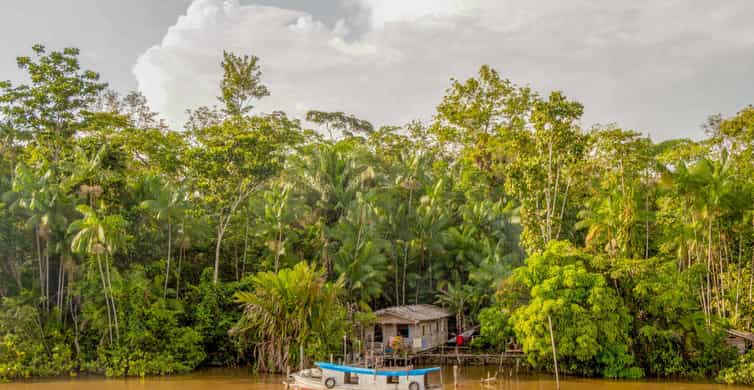The image depicts a tropical, jungle-like setting with dense, lush green vegetation including palms and tall trees, set against a gray, slightly cloudy sky that appears bright. The foreground features muddy, brownish water reminiscent of the Mississippi River or a river in Louisiana. Anchored in the water is a white houseboat with a flat blue roof, equipped with small tires or life savers hanging off its sides. Behind the houseboat, a wooden dock leads up to an old, white wooden structure that resembles a small ranch house or an outpost. This structure is in a state of disrepair, with an open doorway and window frames that are missing their fixtures. The area is totally enshrouded in the dense green vegetation, suggesting a remote, possibly untouched and wild location.